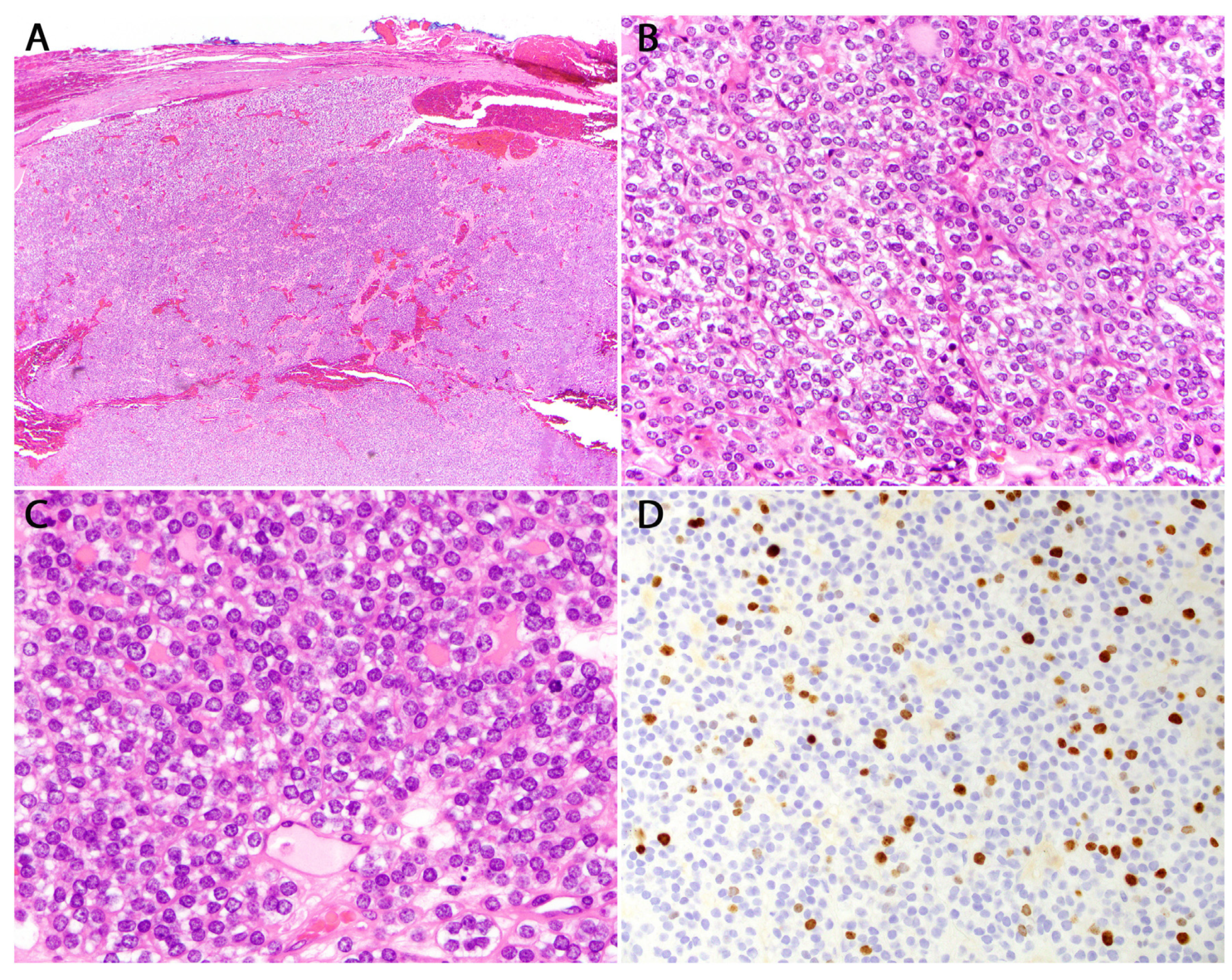The image presents a vivid and detailed microscopic view comprising four distinct sections labeled A, B, C, and D, arranged in a grid formation with A and B on the top row and C and D on the bottom row. Section A features a vibrant fuchsia montage with a mix of purple, white, red, and pink hues, creating a wavy, marbled texture. Section B displays intertwining purple and pink colors with small purple dots along pink lines, resembling cellular structures with a white background. Section C appears as an enlarged version of B, showcasing numerous purple rings and pink splotches against the same white backdrop. Section D differs with a composition of light blue dots scattered throughout, overlaid with brown and dark brown dots on a white background. The overall effect is reminiscent of various microscopic biological samples, illustrating a blend of abstract textures and intricate patterns.